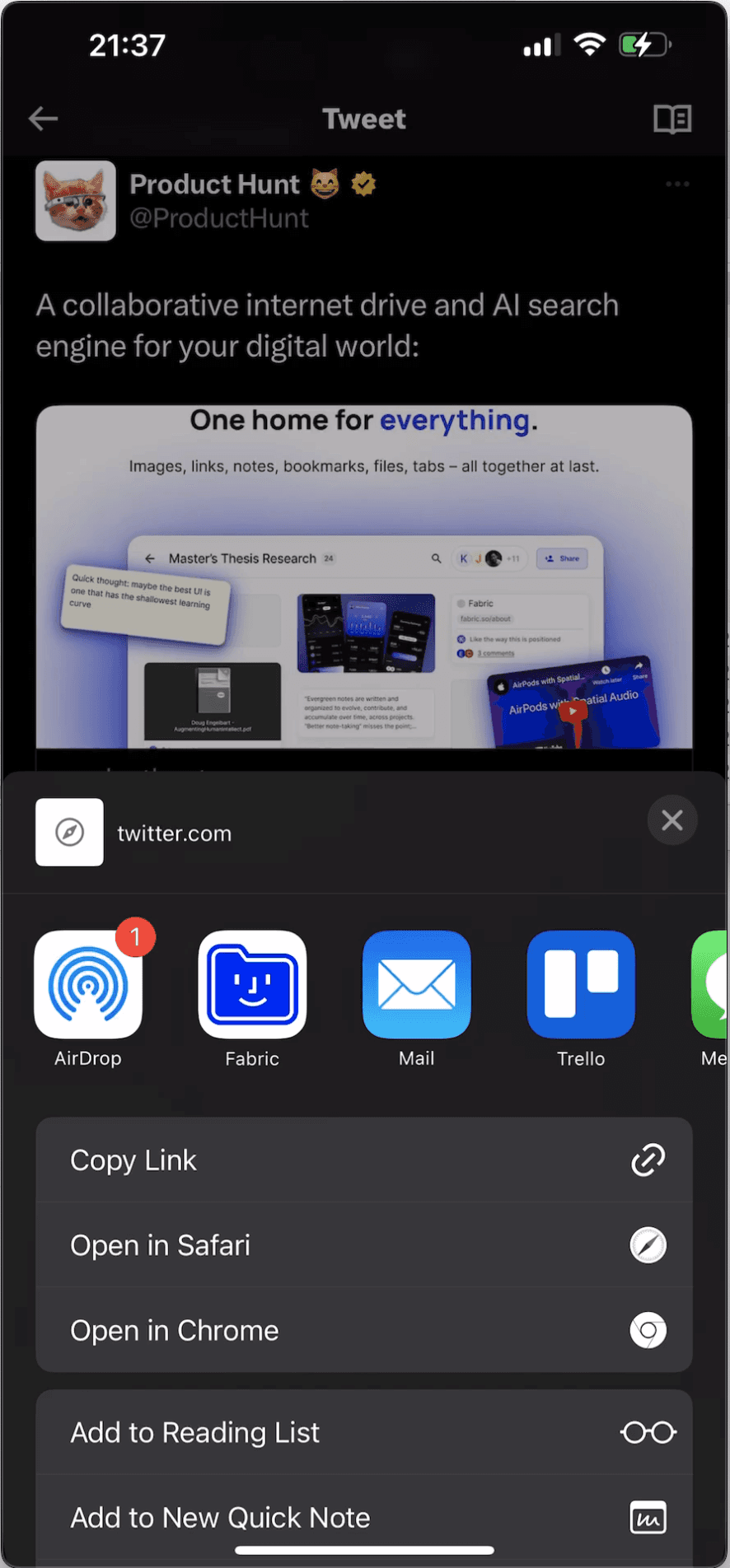Here is a detailed and cleaned-up caption based on the provided description:

---

This image is a screenshot of a cell phone displaying various elements. The top half of the screen has a black background transitioning to a darker gray background midway. In the top left corner, it shows the time as 21:37. In the top right corner, there's a battery icon that is about halfway green, indicating the phone is charging. Next to the battery icon, there is a full Wi-Fi signal symbol followed by three out of four bars, suggesting decent internet connectivity. 

On the left side, a gray arrow points to the left. Centered at the top, it says "Tweet" in white text. On the right side, there is a small open book icon. Below the arrow, there is a white square with a profile picture of a kitty cat wearing sunglasses. To the right of the profile picture, "Product Hunt” is written in white text, accompanied by a kitty cat emoji and a yellow circle with a black checkmark. Beneath "Product Hunt," the username "@ProductHunt" appears in light gray.

The text below describes a product: "A collaborative internet drive and AI search engine for your digital world." Following this, there's a blue section with "One home for everything." in black and blue text. Underneath, it lists features in smaller text: "Images, links, notes, bookmarks, files, tabs - all together at last."

Below this section, a white rectangle showcases phone pictures and text in the top left corner reading "Master Thesis Research." To the left of this, a tab with more text on a white background is shown. In the bottom right corner, an icon resembling a credit card and the text "twitter.com" are visible. Five app icons are displayed at the bottom, with one partially cut off.

At the bottom of the screen, a gray border with white text reads “Copy link,” “Opens in Safari,” and “Open in Chrome.” Beneath that, there's a black bar with white text that says "Add to Reading List" and "Add to Quick Note."

---

This caption provides a comprehensive and coherent description of the screenshot as per the details provided.